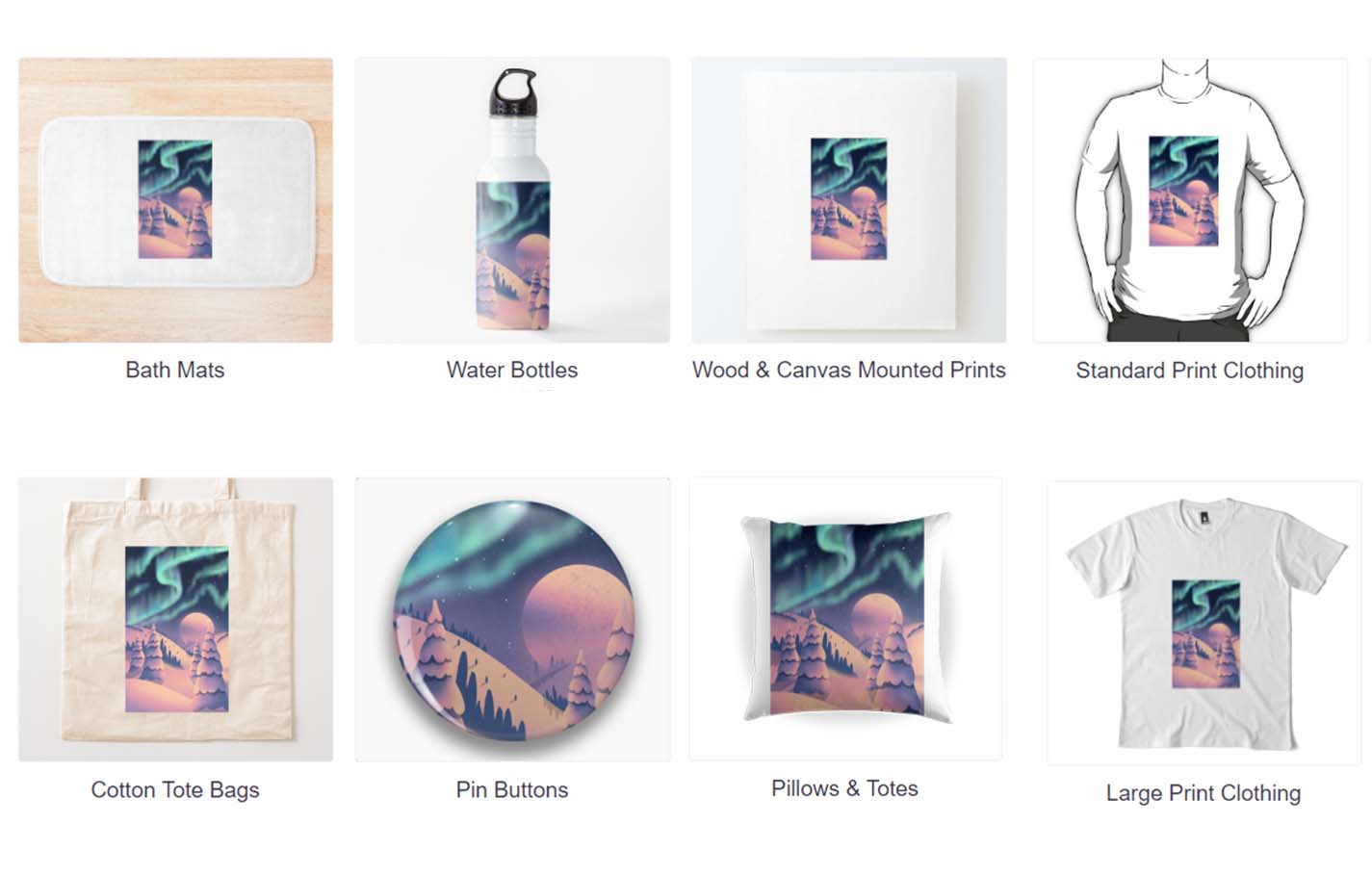Screenshot of a shopping website featuring a grid of eight product images.

In the top row, starting from the left:
1. A bath mat pictured on a light oak-colored plank floor. The product name "Bath Mats" is written underneath in black.
2. A water bottle adorned with a design showing blue squiggles in the sky, an orange moon, and an orange desert landscape. Labeled "Water Bottles" below in black.
3. A wooden canvas-mounted print featuring an identical design of blue squiggles in the sky, an orange moon, and an orange desert with a few dark gray trees. Labeled "Wooden Canvas Mounted Prints" underneath.
4. An illustration of a short-sleeved white shirt showcasing the same blue squiggles, orange moon, and desert image, identified as "Standard Print Clothing" below.

In the bottom row, starting from the left:
1. A cotton tote bag displaying the same design of blue squiggles, orange moon, and desert. The label "Cotton Tote Bags" is underneath.
2. A round button featuring the consistent design. It’s labeled "Pin Buttons" below.
3. A pillow bearing the same recurring image. It’s labeled "Pillows and Totes" underneath.
4. A white t-shirt with a vertical rectangular print of the blue squiggles, orange moon, and desert image positioned on the chest area. It’s labeled "Large Print Clothing" below.